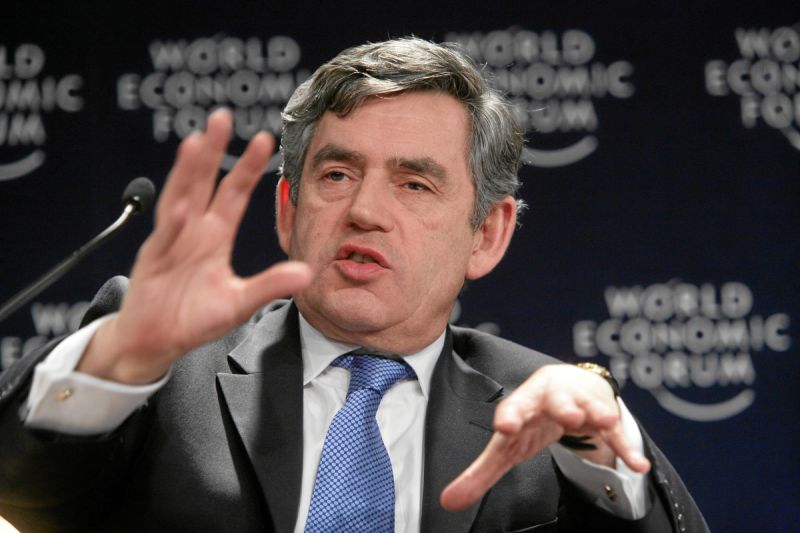This professionally taken photograph captures a man, possibly in his 50s or 60s, speaking at the World Economic Forum. The background prominently features a black wall repeatedly adorned with the white, capitalized text "World Economic Forum." The gentleman, a white male with salt-and-pepper gray hair, is caught mid-sentence with his mouth open and a slight squint in his eyes. He is dressed in a dark gray suit, a white shirt, and a checkered blue and white tie, and wears a watch on his wrist. A microphone is positioned to the left, toward which his right hand gestures, while his left hand is also extended, illustrating his engagement in a significant discussion. The image is rendered in a palette of black, white, various shades of gray, blue, pink, and gold.